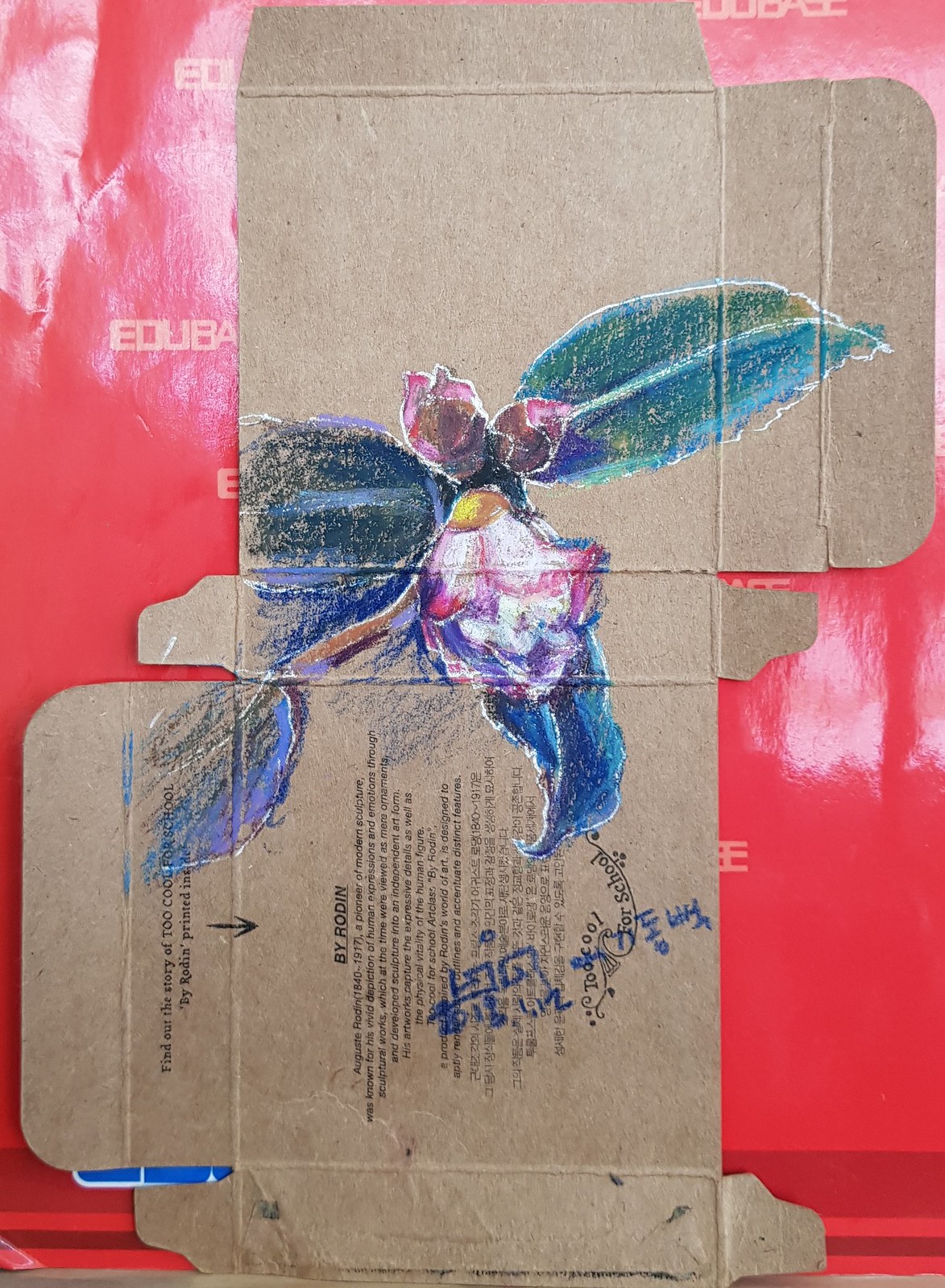This image shows a cardboard box that has been completely unfolded and laid out vertically. The box, which is taller than it is wide, features tabs that have also been folded out, indicating that it was once assembled. The inside of the box is adorned with hand-drawn artwork, depicting a flower in pink and white hues with a yellow center, accented by green and blue leaves. The medium used for the drawing appears to be either crayons or pastels. Additionally, there is text on the box that reads, "By Rodin, Auguste Rodin, a pioneer of modern sculpture, was known for his vivid depiction of human expressions," with the same phrase also written in an Asian language.